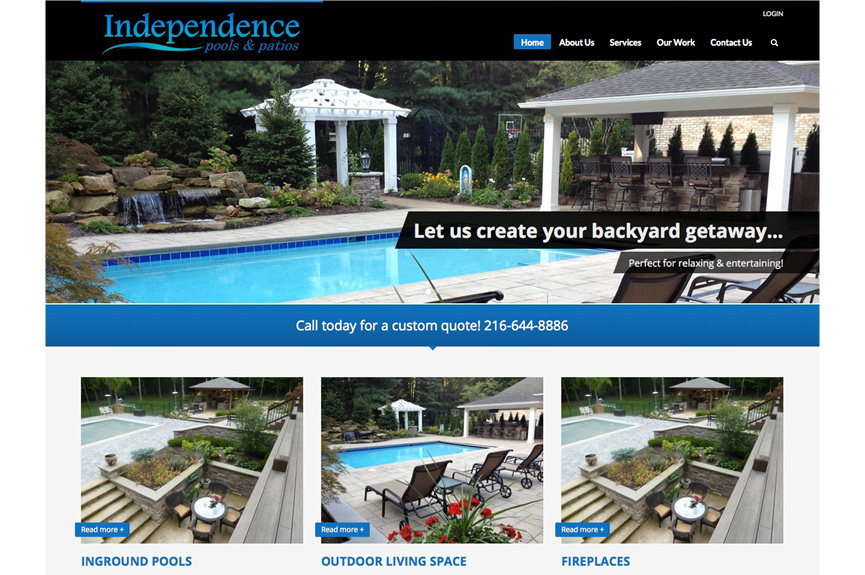The image you're viewing is a snapshot of a webpage from "Independence Pools and Patios." Dominating the site is a panoramic banner image depicting a picturesque backyard oasis. The centerpiece is a sparkling pool surrounded by lush greenery. To the left, a serene water feature adds a touch of tranquility, while on the right, a well-appointed barbecue area with bar stools invites relaxation and outdoor dining. A charming gazebo completes the idyllic scene.

Beneath this main photograph, a prominent blue bar urges visitors to "Call today for a custom quote" at 216-644-8886. Further down, three smaller images align horizontally, each promoting a specialized service: the first image advertises "In-Ground Pools," the second highlights "Outdoor Living Space," and the third focuses on "Fireplaces," with respective pictures illustrating each category.

The descriptive navigation bar at the top of the site offers streamlined links to "Home," "About Us," "Services," "Our Work," and "Contact Us," making it easy for users to explore the offerings of Independence Pools and Patios. The design features cohesive blue text for these categories, ensuring a visually appealing and organized layout.